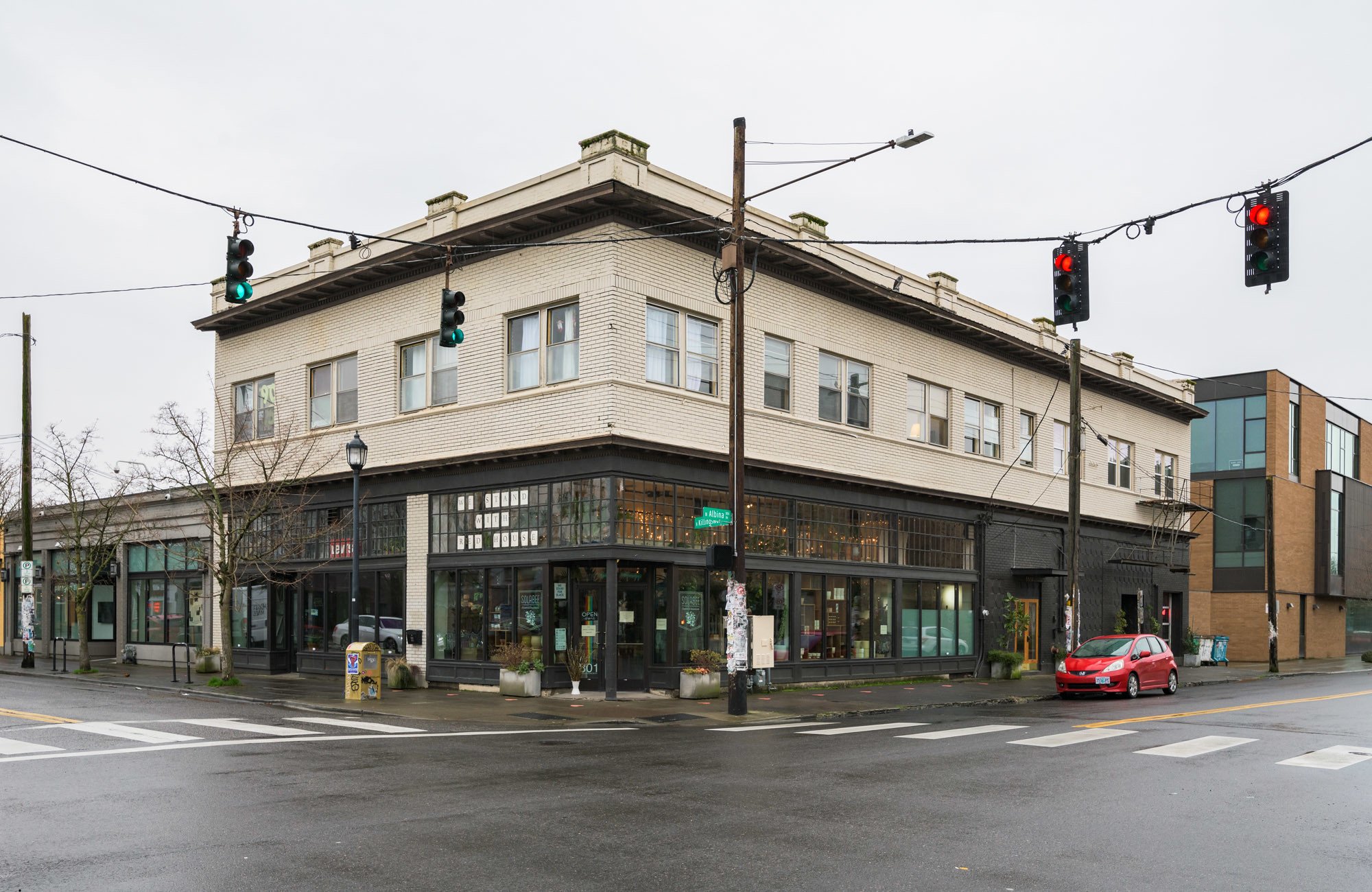The photograph captures a city intersection on an overcast day, where two streets converge at a corner dominated by a notable two-story building. This structure features a white brick upper level, potentially housing commercial offices or living quarters, adorned with numerous windows. The ground level, characterized by dark brown or black panels and surrounded by large plate glass windows with small panes, appears to be a busy retail establishment, possibly a bodega or drugstore. Spanning both intersecting streets, the building fronts are marked by white lettering that remains unreadable. 

Prominently in the frame is a red compact car parked at the corner. The intersection is equipped with older-style traffic lights suspended from cables crossing the streets, with one light showing green and another red. A visible crosswalk delineates pedestrian pathways across both streets, accompanied by a central yellow traffic line. Surrounding the scene are landscape-sized trees on the sidewalks, as well as some silver planters with greenery, contributing to the urban aesthetic. Nearby, occupying the left side of the image, is a shorter, one-story building that appears to be another store, with a yellow structure likely intended for selling newspapers. In the background to the right, stands another brown-bricked building with glass features, adding depth to this urban streetscape bustling with commercial and pedestrian activity. Power poles and lines accentuate the city's electrical infrastructure overhead.